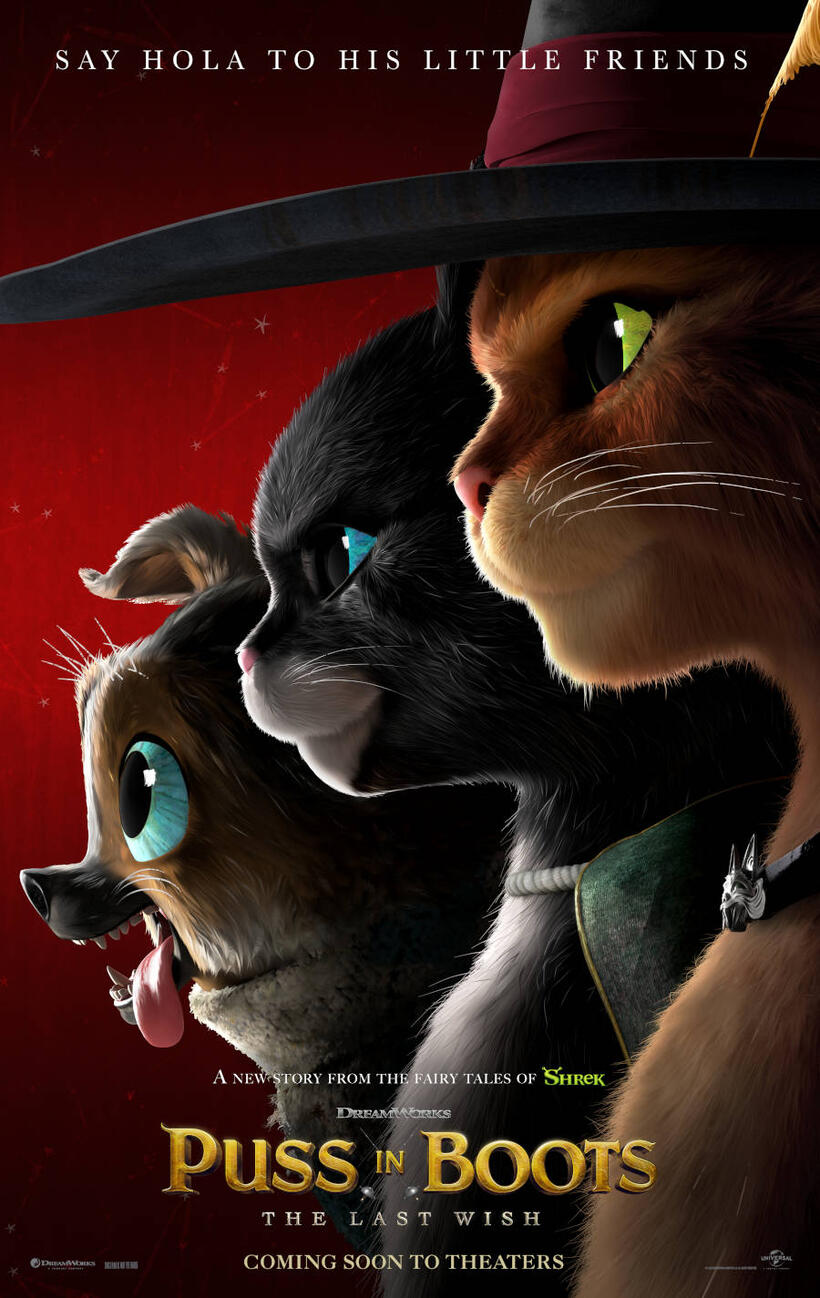This vibrant movie poster for "Puss in Boots: The Last Wish" showcases a striking design with a deep red background that draws your attention immediately. Dominating the scene are the characters' heads and chests, aligned diagonally from the top right to the bottom left. At the top, in bold typography, the poster announces, "Say hola to his little friends," followed by, "A new story from the fairy tales of Shrek." 

The first character is the iconic Puss in Boots, an orange tabby with piercing green eyes, sporting his signature black hat adorned with a red band and a yellow-orange feather. Below him is another cat, a black feline with a striking blue eye and a distinctive necklace. Completing the trio is a playful dog with one blue eye, showcasing sharp teeth and a tongue hanging out. 

The bottom of the poster details the film's title, "DreamWorks Puss in Boots: The Last Wish," and notes, "Coming soon to theaters," promising an exciting new adventure in the beloved Shrek universe.